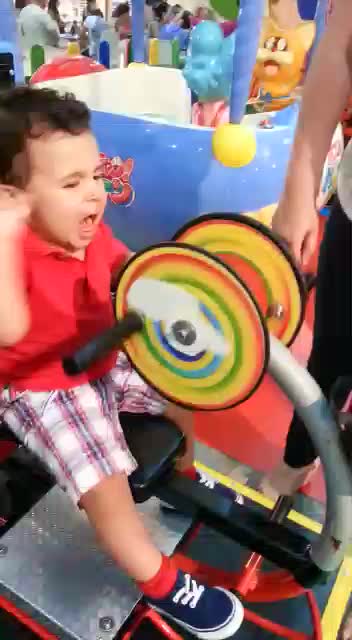In the vibrant image, a young child, approximately two years old, sits on a colorful ride with handlebars and a seat, suggesting it might be a playful vehicle or toy. The child is strikingly dressed in a red polo shirt, white shorts with stripes, red socks, and blue shoes with white laces. His dark, possibly curly, hair adds to his expressive demeanor as he looks straight ahead, his mouth open and eyes narrowed, almost forming a fist with his hand, hinting at a moment of distress or determination.

Surrounding him, there are elements of a lively, fun event, potentially a carnival, evidenced by various cartoon-like structures that evoke a theme park feel, similar to those at Chuck-E-Cheese. Notably, in the background, a light baby blue teapot ride enhances the playful atmosphere with its soft pastel colors. An adult’s arm, likely his mother's, is visible beside him, adding a touch of guardianship in the child-centric setting. The ride itself has vibrant, spiral designs that may create a hypnotic effect when spun, further enriching the whimsical scene.